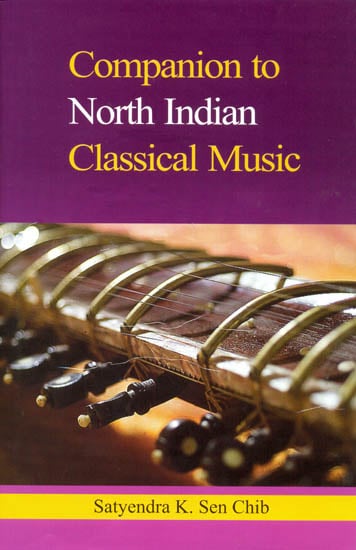The image appears to be a scan of a book cover titled "Companion to North Indian Classical Music." The book is authored by Satyendra K. Senchib. The title is prominently displayed at the top with "Companion to" in yellow text, "North Indian" in white, and "Classical Music" back in yellow. Below the title, there is a central photograph of a musical instrument, which looks like a sitar, featuring a mix of brown and silver with black knobs. The name of the author, Satyendra K. Senchib, is written in a dark font against a yellow stripe that spans the width of the cover. The background is primarily pink with a dark purple area above the title. Overall, it has the appearance of a conventional book cover designed to convey information about North Indian classical music.